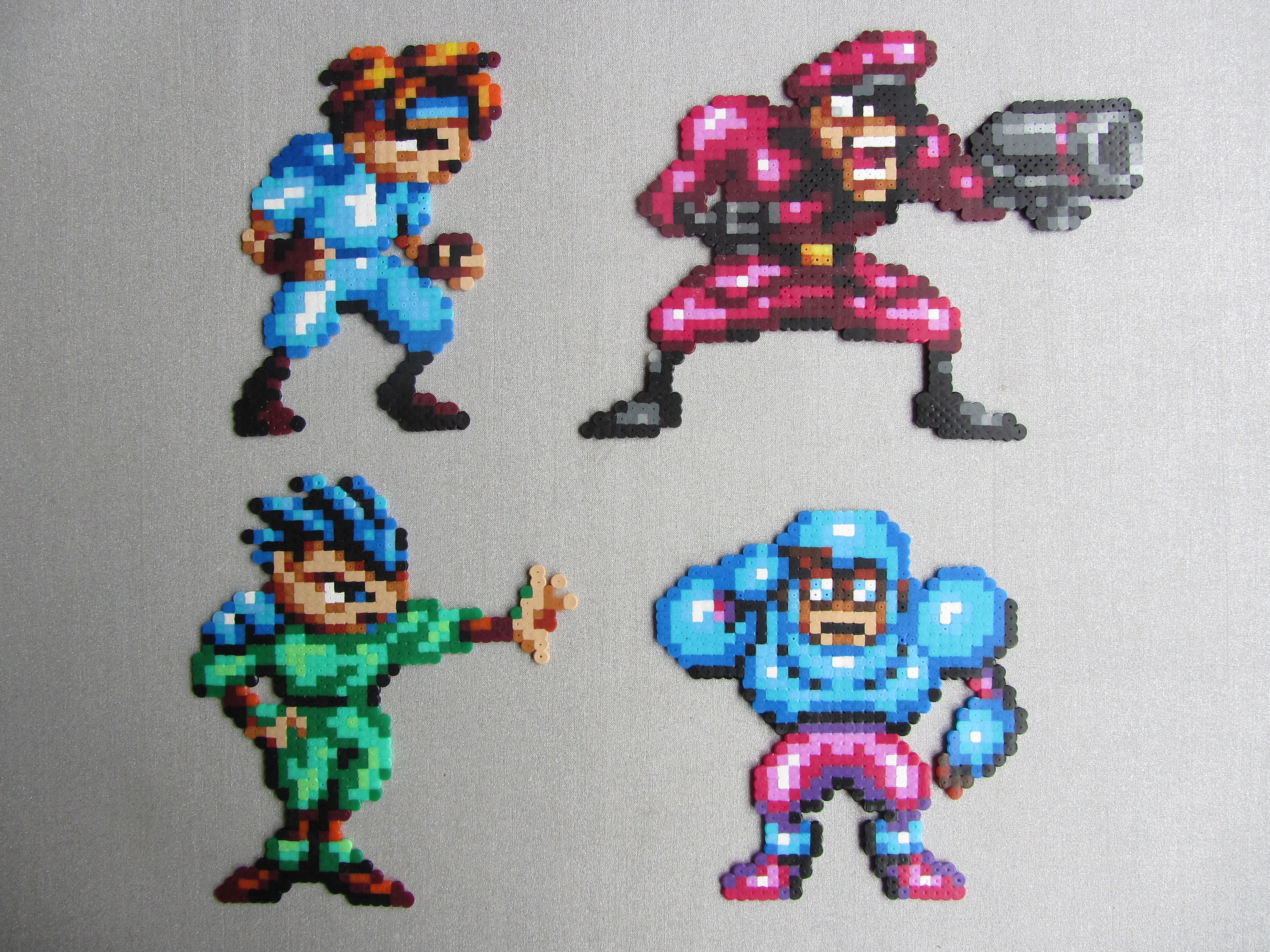The image is a blurred photograph of four pixel art decals resembling characters from a video game, possibly akin to those from Mega Man, affixed to a gray, cloth-like background. Arranged in a square with two figures on the top and two on the bottom, each character is composed of large, colored dots, providing a 3D feel. 

In the top left, there's a Caucasian male fighter, donning a blue outfit with a matching headband, brown hair, and black boots. His hands are clenched into fists as if ready to brawl. To the right, a character resembling a military commander stands, dressed in a red skin suit and black boots, holding a blaster in his left hand. He has an eyepatch over his left eye and his mouth open in a shout, mirroring Major Bison from Street Fighter.

On the bottom left, another fighter in a green suit with brown boots and a blue shoulder pauldron is depicted. This character sports spiky black hair with blue highlights, extending his left hand as if to unleash an attack. Lastly, on the bottom right, a figure in a space suit is seen, characterized by a blue top half, pink pants, and blue and pink boots. This individual wears glasses with a raised right hand in a salute, while the left hangs to the side. All four figures are blurred but detailed enough to convey their distinct video game-inspired designs.